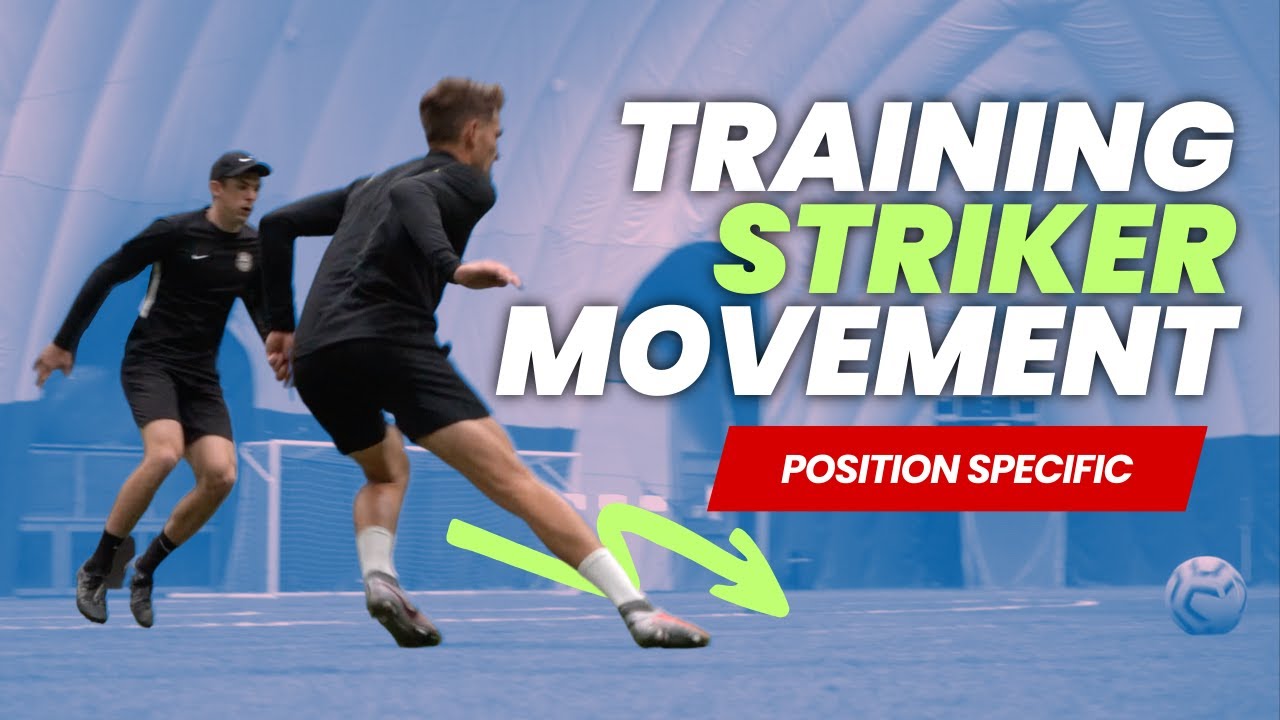The image is a poster or thumbnail for an instructional soccer video or course. It prominently features the text "Training Striker Movement" with "training" in white, "striker" in light green, and "movement" in white again. Below this, in a red banner with white letters, it states "Position Specific." The poster shows two men on an indoor soccer pitch with a blue-shaded background and an inflatable dome roof. Both men are in black shirts and shorts; one has black socks, while the other has white socks. One player wears a cap. They are both focused on a soccer ball situated in the lower right corner of the image. Yellow arrows point from the knee of the player on the right toward the pitch, indicating the directions for "striker movement." Behind them, a soccer net is visible in the center background, against the blue-toned setting.